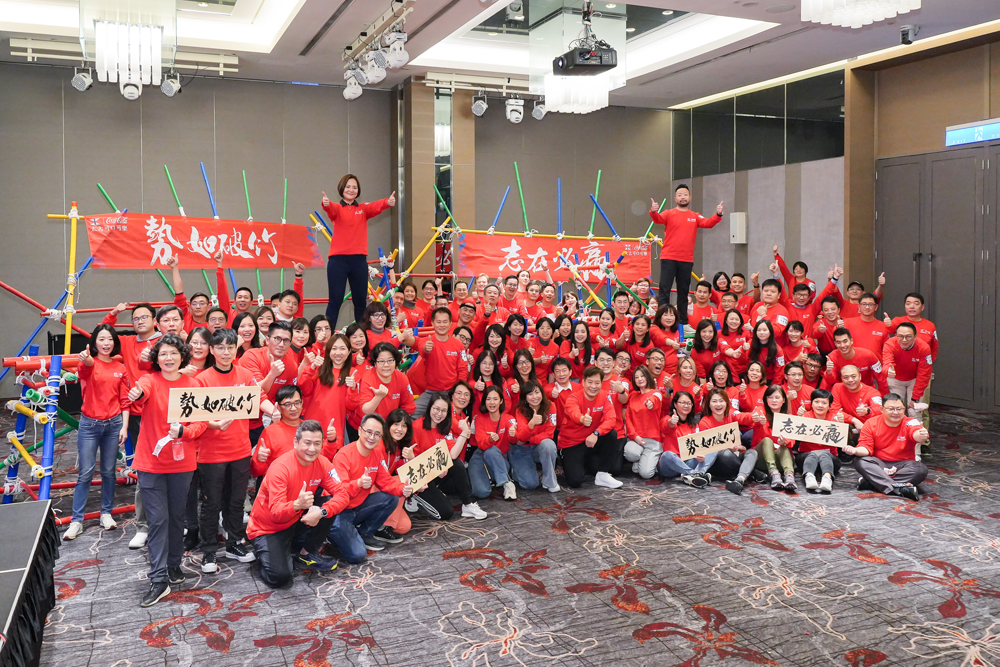The image captures a large group of around 80 to 100 people, all dressed in identical red shirts emblazoned with an unreadable logo, gathered for what appears to be a formal group photograph inside a spacious, hotel ballroom-like venue. The room, illuminated by overhead lights including some spotlights and a ceiling projector, features gray carpeting accented with maroon or red patterns and floral outlines. The background is marked by several banners with Asian script, possibly Chinese, flanked by two individuals standing with outstretched arms on either side, presumably group leaders. The group is arranged in roughly four rows: the front row seated on the floor, the middle rows either standing or crouching, and the backmost rows elevated on platforms or scaffolding. Some additional details include lockers and windows on the far right, and the edge of a table in the lower left corner of the photo. The participants, dressed variably in dark pants and even a pair of white pants, appear cheerful and united for the photograph.